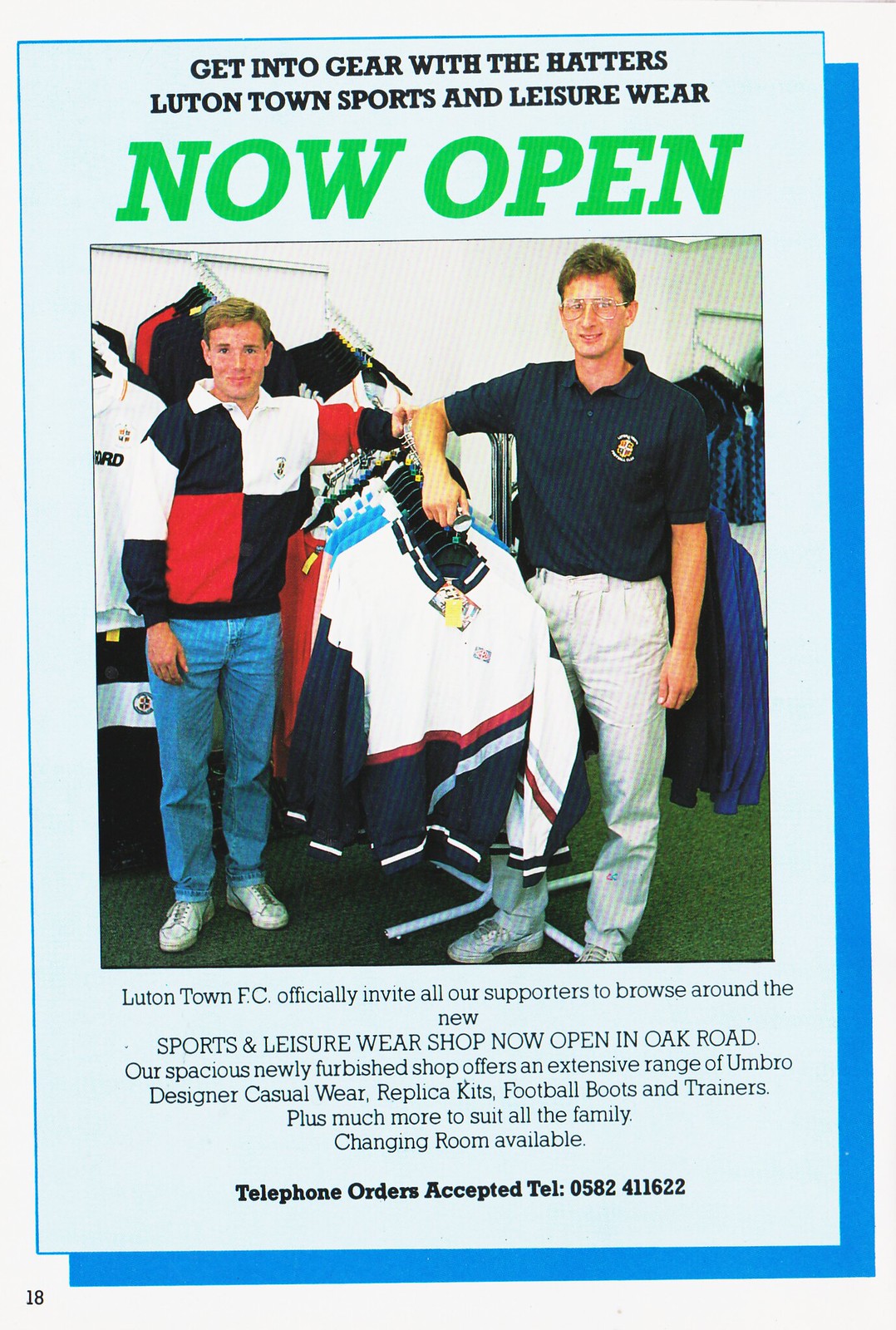**Get into Gear with the Hatters: Luton Town Sports and Leisure Wear Now Open**
 
This vintage magazine advertisement features Luton Town FC's sports and leisure wear shop in Oak Road. The ad is designed with a sky-blue background framed by a darker blue shadowed border, creating a striking visual appeal. At the top of the ad, in bold black uppercase letters, it reads: "Get into Gear with the Hatters, Luton Town Sports and Leisure Wear." Immediately below, in bold green italic letters, the ad announces: "Now Open."

The centerpiece of the advertisement is a tall rectangular photograph of two men standing in front of rows of hanging sports jackets. The man on the left, a white man with blonde hair, is dressed in a long-sleeved polo shirt featuring a black, white, and red square pattern, blue jeans, and white sports shoes. The man on the right, also a white man, wears glasses and is dressed in a blue short-sleeved polo shirt with a logo on the left chest, white pants, and white sports shoes. The jackets hanging behind them are primarily white with blue sleeves accentuated by red and white lines. Below the photograph, the text reads: "Luton Town FC officially invite all our supporters to browse around the new Sports and Leisure Wear shop now open in Oak Road." Additional details highlight the shop's offerings of Umbro designer casual wear, replica kits, football boots, trainers, and more to cater to all family members. At the bottom left corner of the ad, the page number "18" is visible, and a footnote states: "Telephone orders accepted. Telephone 0582-411-622."

This detailed and well-organized advertisement effectively captures the new store's grand opening and extensive product range, inviting Luton Town FC supporters to visit and explore.